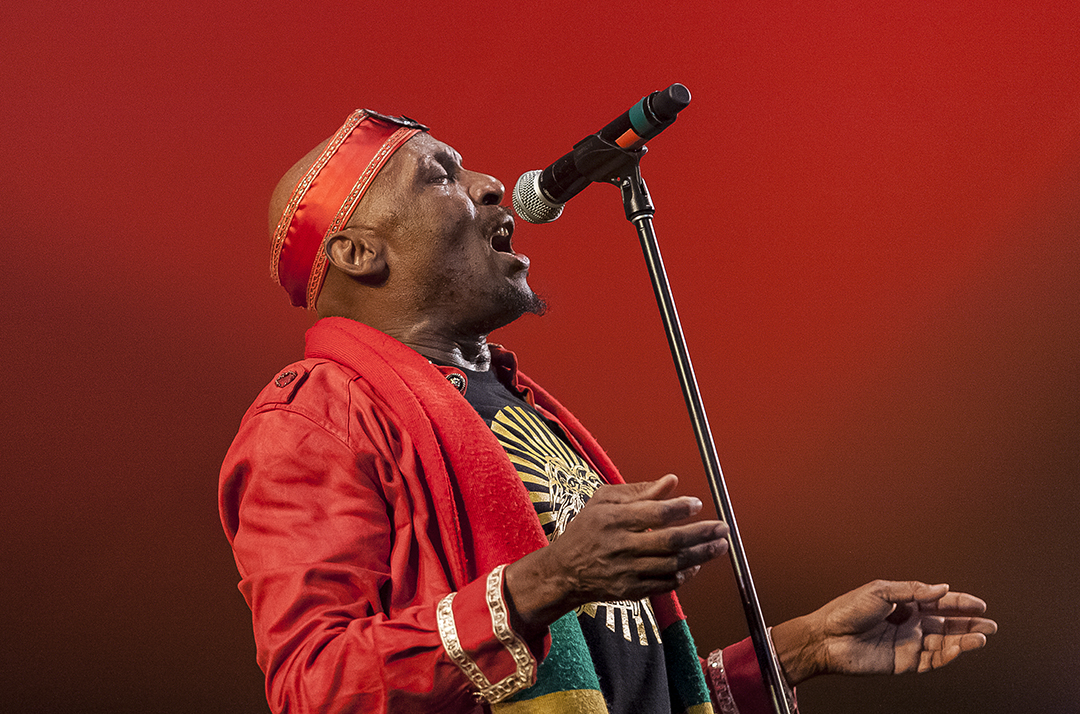The photograph captures a man passionately singing on stage, focusing on him with a shallow depth of field that contributes to the dramatic effect. The man sports a shaved head adorned with a red headband and has a small goatee and mustache. His mouth is open and his eyes closed as he sings into a black microphone fixed on a stand positioned to his right. He is dressed in a striking ensemble consisting of a vivid red coat over a black T-shirt adorned with a golden symbol in the center. Draped around his neck is a shawl, predominantly red with touches of blue and yellow at its corners. The background is a vivid, grainy red that darkens to almost black towards the bottom, likely due to a combination of stage lighting and smoke effects, enhancing the overall intensity of the scene.